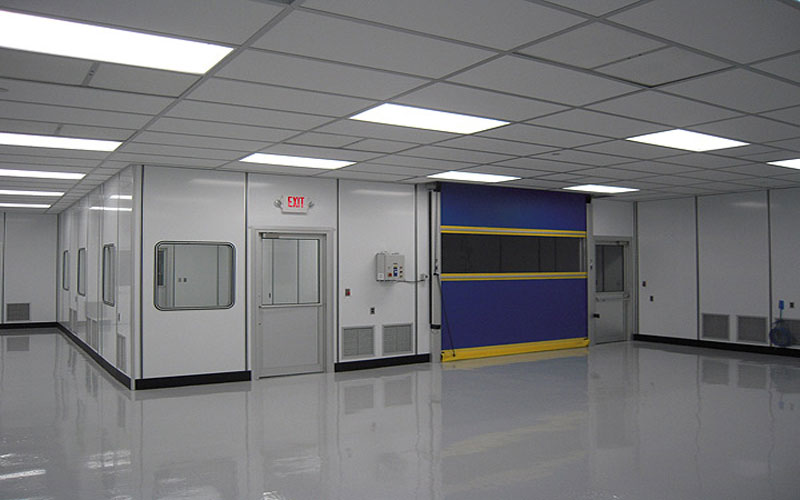The image depicts the interior of a sterile, industrial-looking building. The room is empty and characterized by its white, shiny, and meticulously clean floor, which gives off a buffed appearance. The walls are predominantly white, segmented by silver metal panels. Overhead, a grid system of tile panels with fluorescent lighting illuminates the space evenly. 

In the center of the room, there is a structure reminiscent of two smaller rooms within the larger room. One of these doors has a red exit sign above it, with three side windows flanking it to the left and one window in the front. Nearby, an electronic device is mounted on a box attached to the wall. Adjacent to this is another door with a distinct design: it features a variety of horizontal stripes in navy blue, yellow, and black, resembling a garage door. This door area is outlined by slivers of navy blue and bordered by yellow and black stripes in varying thicknesses. 

An additional silver door with an exit sign overhead is positioned to the left of this elaborate door. A bench runs along the bottom of the wall panels, adding to the industrial aesthetic. Grates and vents are present in the walls, providing airflow. The overall impression is one of a clinical, highly maintained environment, possibly used for industrial or technical purposes.